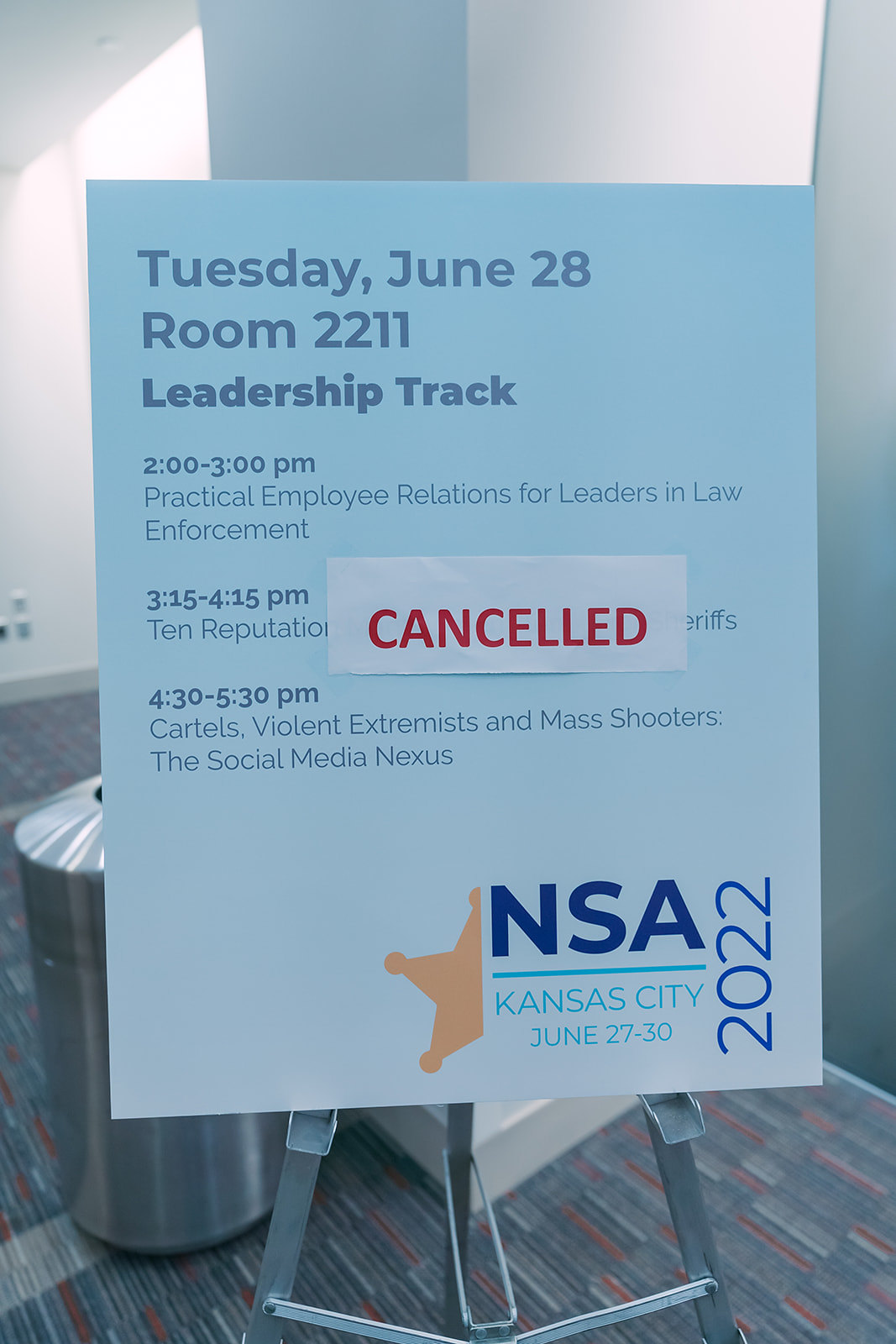The poster, mounted on a metal easel, features a blue background with darker blue and white text. At the top, large letters announce: "Tuesday, June 28th, Room 221, Leadership Track." Below, it outlines the event schedule:

- 2 to 3 p.m., "Practical Employee Relations for Leaders in Law Enforcement."
- 3:15 to 4:15 p.m., "Reputation..." (partially obscured by a white piece of paper with "Canceled" in red text).
- 4:30 to 5:30 p.m., "Cartels, Violent Extremists, and Mass Shooters: The Social Media Nexus."

In the bottom right corner, the poster mentions "NSA, Kansas City, June 27th to 30th, 2022" alongside a half gold star. The surrounding environment includes a silver metal trash can, a striped carpet with red, black, gray, and white stripes, and white walls.